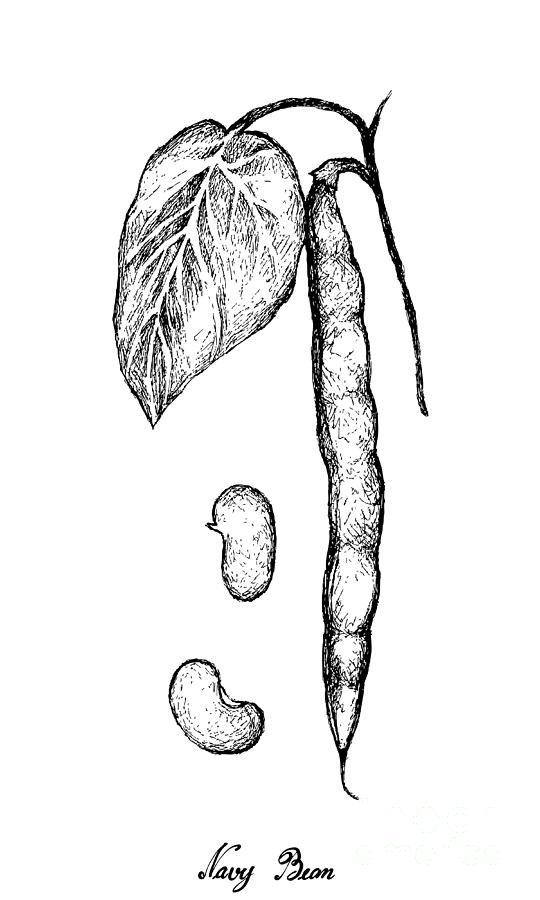This is a detailed black and white ink drawing of a navy bean plant. The illustration features a prominently centered bean pod with a textured stem and a large, detailed leaf, revealing the intricate veins. At the bottom of the sketch, in cursive script, is the label "Navy Bean." The drawing skillfully captures the ribbed appearance of the bean pods, which contain about four to five beans, emphasizing the plant's natural form. Next to the main pod are two individual beans, providing a clearer view of their shape. The image relies on shading to add depth and intricacy, presenting a textured and almost charcoal-like finish. No colors are used, and no other objects or text appear, making the navy bean plant the sole focus of this detailed monochromatic artwork.